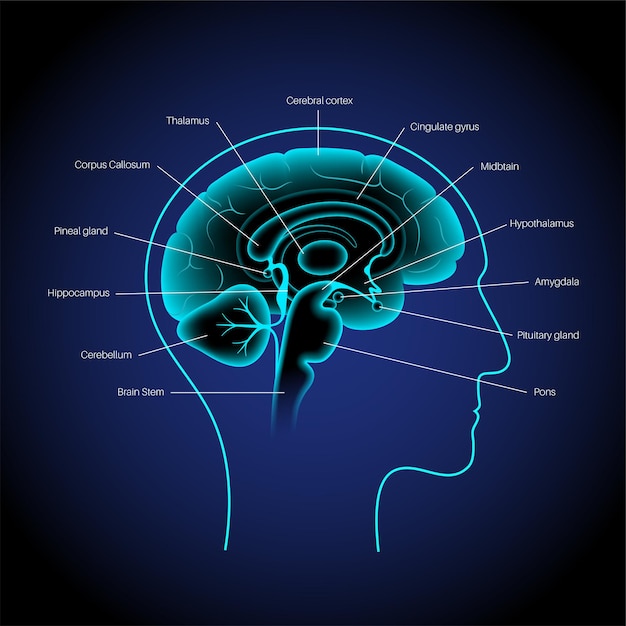This detailed color illustration features a silhouette of a human head in profile, delineated by a light teal blue line against a square backdrop that transitions from a black gradient around the edges to a darker blue near the center. The inside of the head reveals a brain, outlined in blue with a gradient from light aqua around the edges to black in the center, and highlighted with aqua to define various brain structures. White lines radiate from the circumference of the head, each pointing to specific labeled parts of the brain. From left to right, these labels identify the brainstem, cerebellum, hippocampus, pineal gland, corpus callosum, thalamus, cerebral cortex, cingulate gyrus, midbrain, hypothalamus, amygdala, pituitary gland, and pons. The overall style combines elements of text and graphic design to create an educational and visually engaging representation of the human brain.